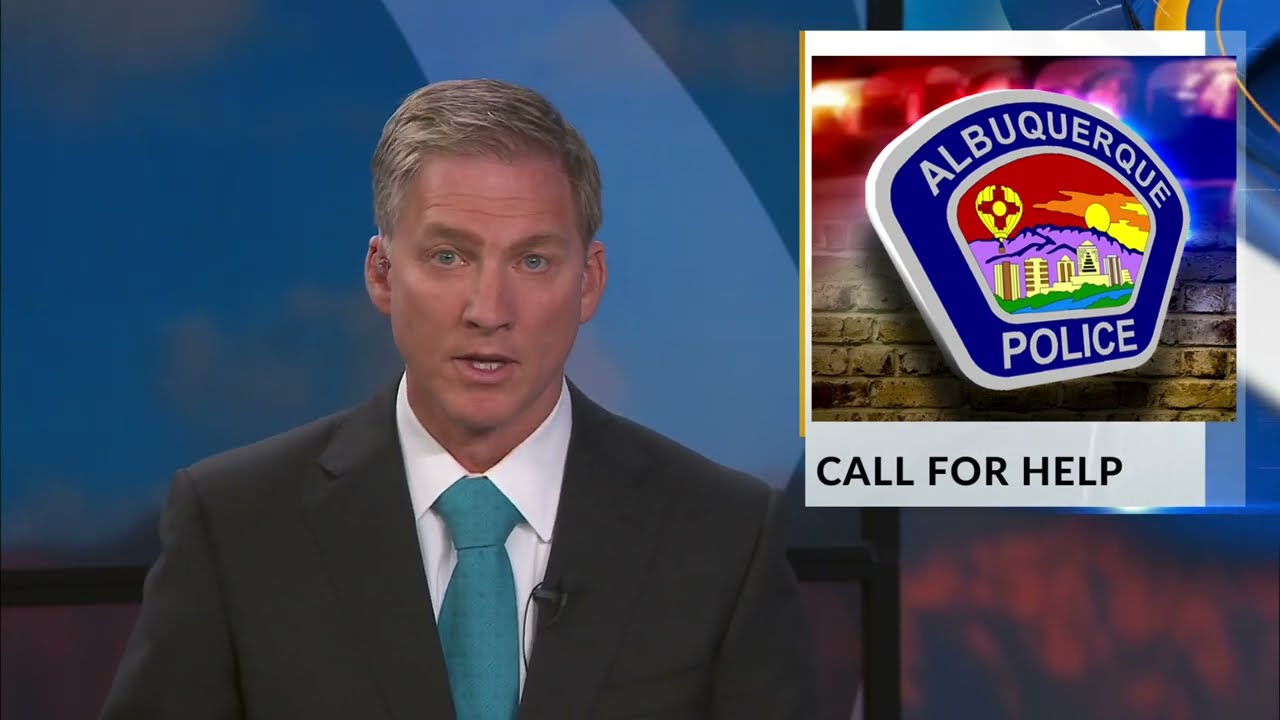A middle-aged news anchor, likely in his 40s or 50s, is pictured sitting and speaking towards the camera. He has dirty blonde hair, blue eyes, and a tanned complexion. Dressed in a dark gray suit jacket, a white button-down shirt, and a turquoise tie featuring a small geometric pattern, he also wears an earpiece in his right ear and a microphone attached to his lapel. His mouth is slightly open as if he’s in the middle of delivering a report. The background is a blend of blue and orange with a curved lighter blue section that mimics a window setup. In the upper right corner of the image, there is a graphic featuring an Albuquerque Police badge, appearing in a computerized style. Below the badge, in a white box with black all-capital letters, is the text "CALL FOR HELP."